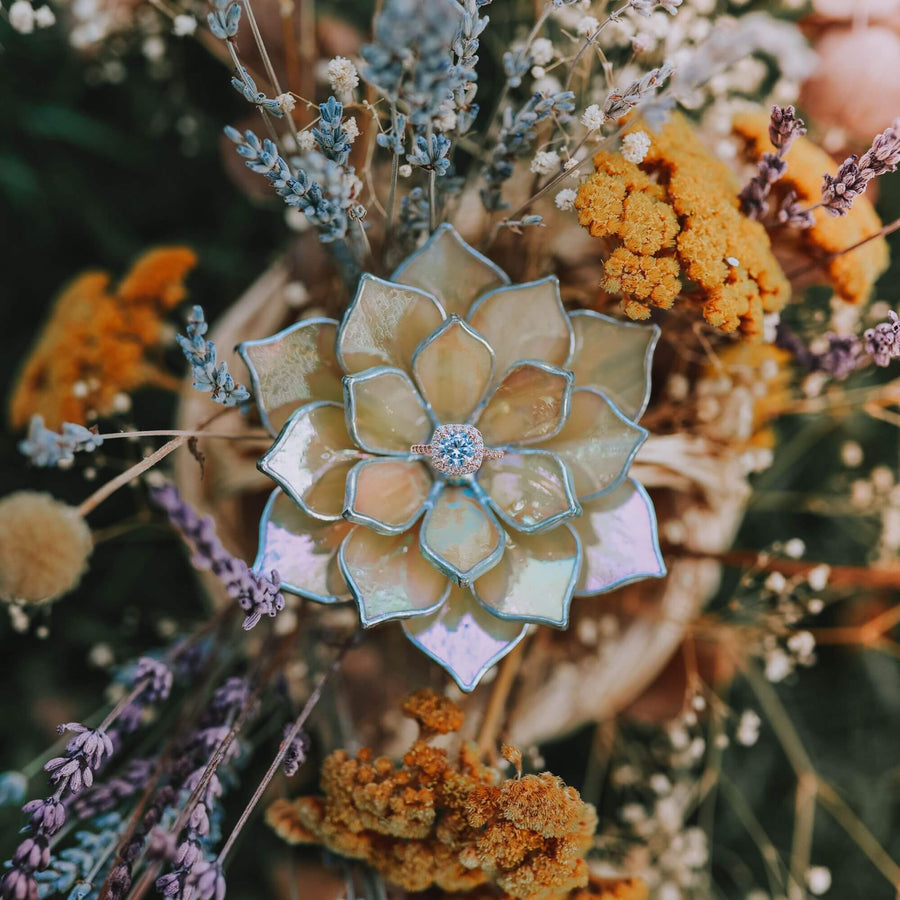This image shows a top-down view of an intricate decorative arrangement, featuring a centerpiece that appears to be an artificial, glass-like flower. This central flower, resembling a combination of marble and stained glass, radiates with silvery, beige, and light gold petals that boast a sparkling texture. The middle of this flower is particularly striking, containing a square, jewel-like element with a blue hue that mimics the appearance of an engagement ring. Surrounding this focal point are a variety of smaller, artificial flowers in vivid shades of blue, purple, and orange, contributing to the arrangement's vibrant fall palette. Additionally, there are tiny, blurry white flowers located in the bottom right and top left corners, accompanied by dark grass-like plants. The overall effect is a stunning, almost mosaic-like composition, where the central flower is in clear focus, while the surrounding elements create a harmonious but slightly out-of-focus backdrop.